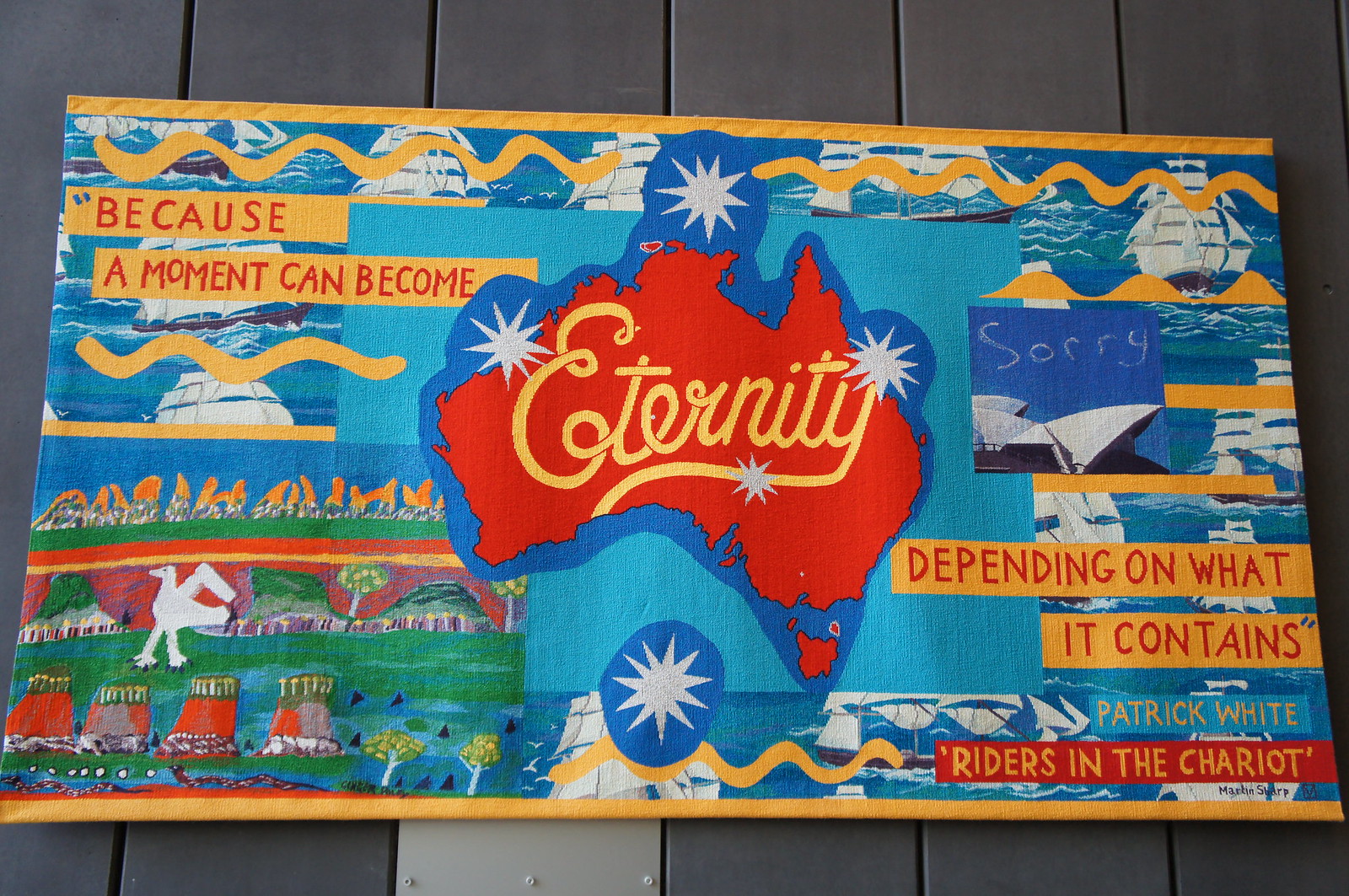This image is a vibrant and colorful poster mounted on a wall with grey wooden paneling, featuring both dark and light grey slats. Dominating the center of the poster is a striking red map of Australia, bordered in blue with white sun shapes scattered across it. Prominently overlaying the map in yellow script is the word "Eternity." The poster is vivid, incorporating bright hues of blue, yellow, and green throughout its design. Around the border, various phrases are inscribed in alternating red font on a yellow background and yellow font on a red background. Key phrases include "Because the moment can become eternity depending on what it contains," and "Patrick White, Riders in the Chariot." Additionally, the poster features multiple images, such as the Sydney Opera House with the word "Sorry," sailboats, birds, rock formations, trees, and mountains, adding to the visual richness. This piece blends artistic elements with textual details, creating a kaleidoscopic and thought-provoking visual narrative.